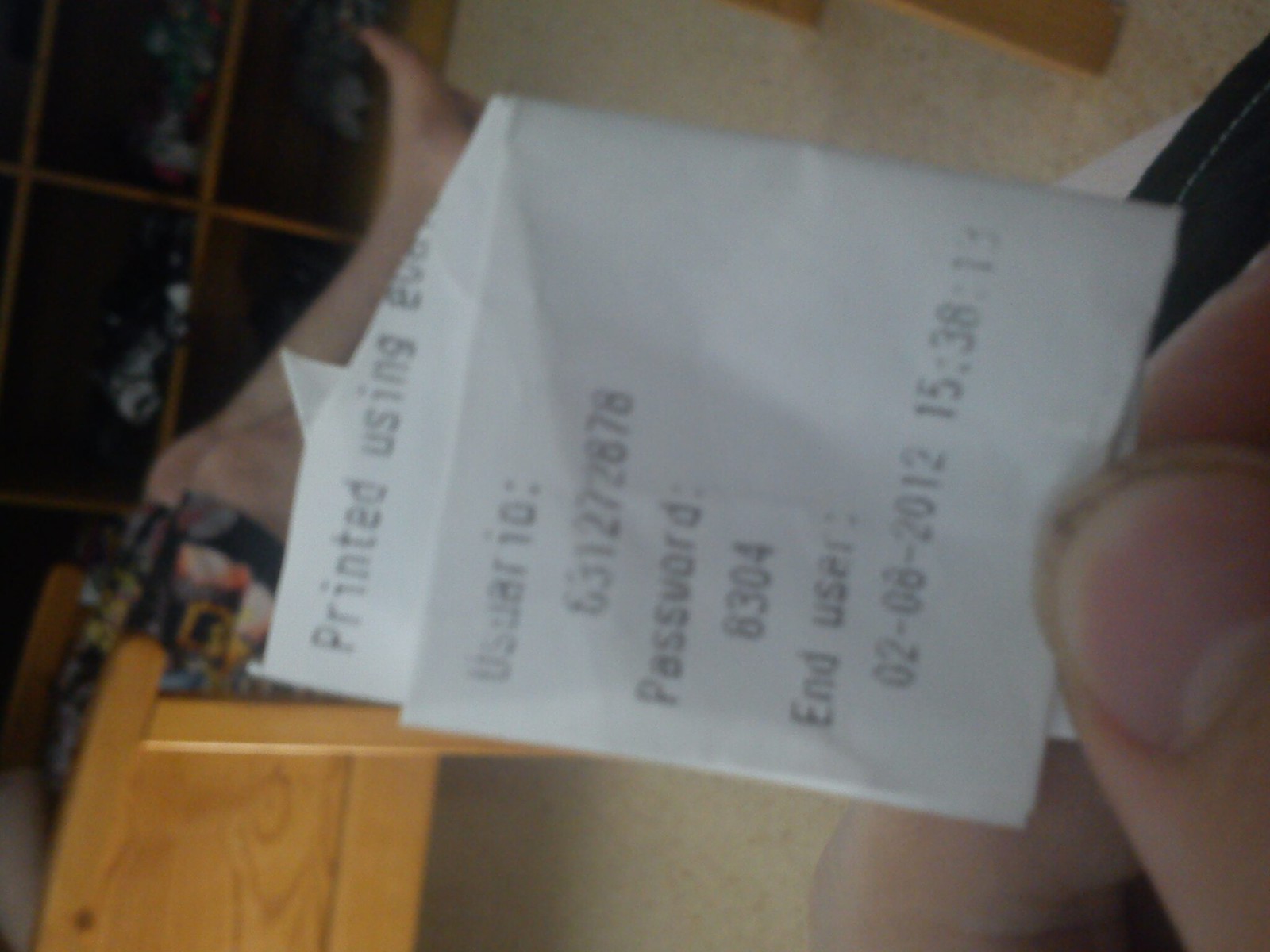In the image, the thumb and index finger of a Caucasian individual are holding a white, slightly folded receipt. The receipt contains a user ID, a sequence of numbers "631272878," and a password "8304." Additionally, the receipt mentions an end user date "02-08-2012," paired with a military time "15:38:15." The background reveals another Caucasian individual seated on a brown wooden chair. The setting features a beige carpet, adding a neutral tone to the scene. The image captures the intricate details of the receipt along with elements of the surrounding environment, providing a snapshot of a precise moment.